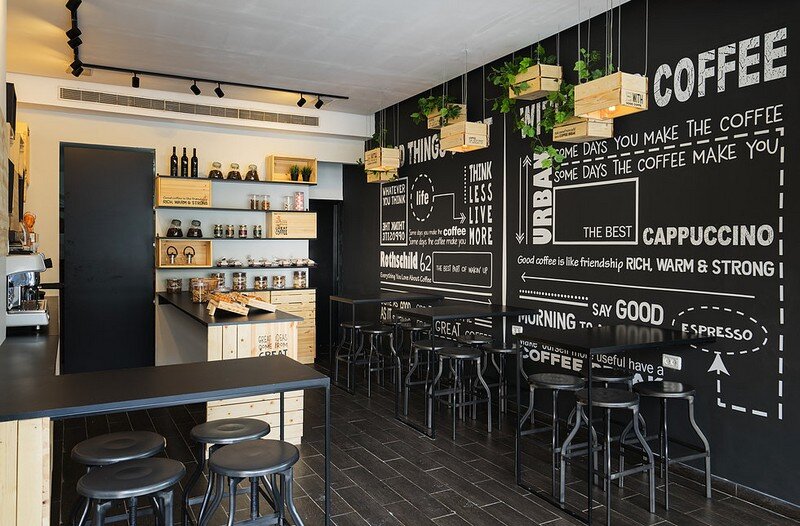The photograph captures a modern, industrial-style coffee shop. The focal point is a black wall adorned with various white text, featuring sayings like "the best cappuccino" and "good coffee is like friendship, rich, warm and strong." Along this wall, three tables are set up with dark gray or black metallic stools. Hanging from the ceiling are wooden flower pots and unique rectangular lamps with light bulbs inside, suspended by thin wires. 

On the left side of the image is a countertop holding a coffee machine, suggesting a functional kitchen area with shelves filled with wine bottles and jars. Studio lights are affixed to the ceiling, casting a bright, heavy light, especially from the front right side of the shop. The rightmost section of the photograph shows multiple tables lined with stools, emphasizing the inviting, communal atmosphere of the space.